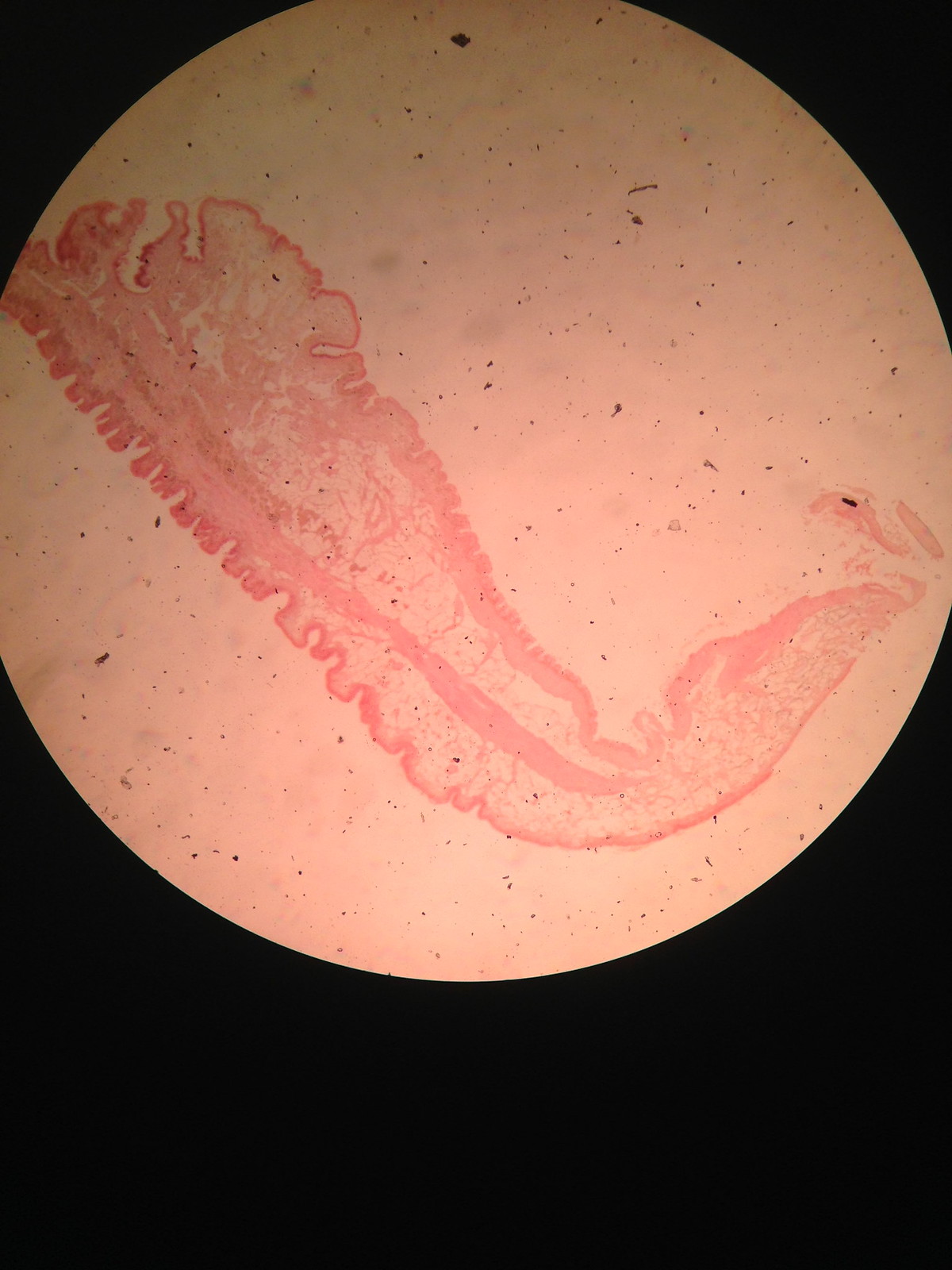The image depicts a circular, pinkish medical slide set against a black background. At its center is a light pink, slightly transparent, and curved structure that closely resembles tissue or a thin slice of muscle viewed under a microscope. This central structure features intricate details such as red, vein-like patterns and small capillary-like designs, suggesting it could be part of an organ. Surrounding this main blob, the background is scattered with various black and pinkish dots, adding an abstract, cluttered effect to the image. The overall appearance evokes the texture and complexity of biological tissue, hinting at a highly magnified view of cellular or muscular components.